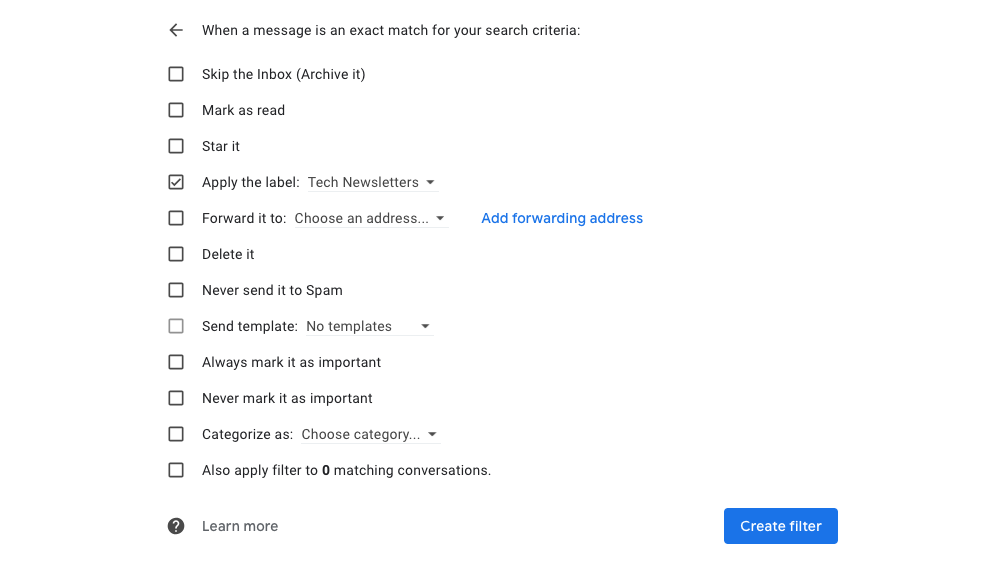Screenshot of an email filtering rule setup:

The screenshot captures a white-background interface inside an email client where filtering rules are being configured. It states: "When a message is an exact match for your search criteria."

The primary focus is a list of actions that can be applied to matching emails, where the first option, "Skip the inbox (Archive it)," is checked. Further down the list, the following actions are displayed, with specific details noted:
- "Mark as read" (unchecked)
- "Star it" (unchecked)
- "Apply the label: Tech newsletters" (checked)
- "Forward it to" (with no email address filled)
- "Delete it" (unchecked)
- "Never send it to Spam" (unchecked)
- "Send template" (unchecked)
- "Always mark it as important" (unchecked)
- "Never mark it as important" (unchecked)
- "Categorize as" (option not selected)
- "Also apply filter to 0 matching conversations" (unchecked)

Towards the bottom of the interface, there's a question mark icon inside a black circle, labeled "Learn more." Finally, a blue box at the bottom of the screenshot displays the button "Create filter," which, when clicked, will apply the chosen action to future emails that match the specified criteria.

In summary, the primary action to be applied is to "Apply the label: Tech newsletters," indicating that any email meeting the exact search criteria will automatically be labeled under "Tech newsletters."